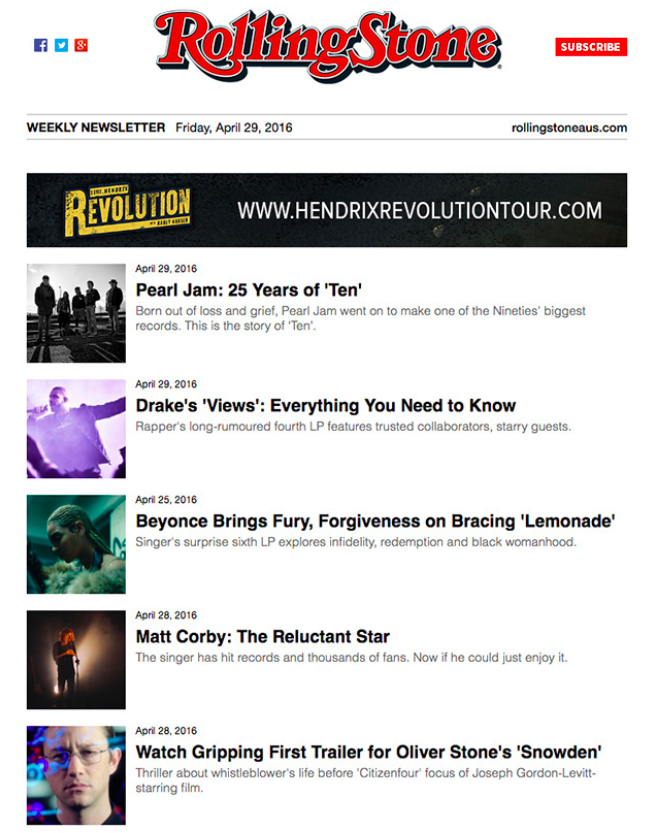In this image, we see a detailed screenshot from the Rolling Stone website.

At the very top, "Rolling Stone" is prominently displayed in dark red letters with black outlining. To the right of this logo, there is a red "Subscribe" button with white text, accompanied by three social media icons.

Just below this header, the screen shows information about the "Weekly Newsletter" dated Friday, April 29, 2016, and to the right of this, RollingStoneUS.com is listed. Further down, there is a heading "Revolution" in gold text, followed by the URL www.HendrixRevolutionTour.com in white text against a black background.

The lower section of the screenshot features five headlines, each accompanied by dates and brief descriptions:

1. **Headline: "Pearl Jam: 25 Years of Ten"**
  - Date: April 29, 2016

2. **Headline: "Drake: Views – Everything You Need to Know"**
  - Date: April 29, 2016

3. **Headline: "Beyoncé Brings Fury and Forgiveness on Bracing Lemonade"**
  - Date: April 25, 2016

4. **Headline: "Matt Corby… The Reluctant Star"**
  - Date: April 28, 2016

5. **Headline: "Watch Gripping First Trailer for Oliver Stone’s Snowden"**
  - Date: April 2016
  - An image of each character from the trailer appears to the left of this headline.

The entire lower portion of the webpage presents these headlines and dates against a white background, providing a clean and organized look. The formatting and color schemes distinguish each section clearly, maintaining a user-friendly interface.